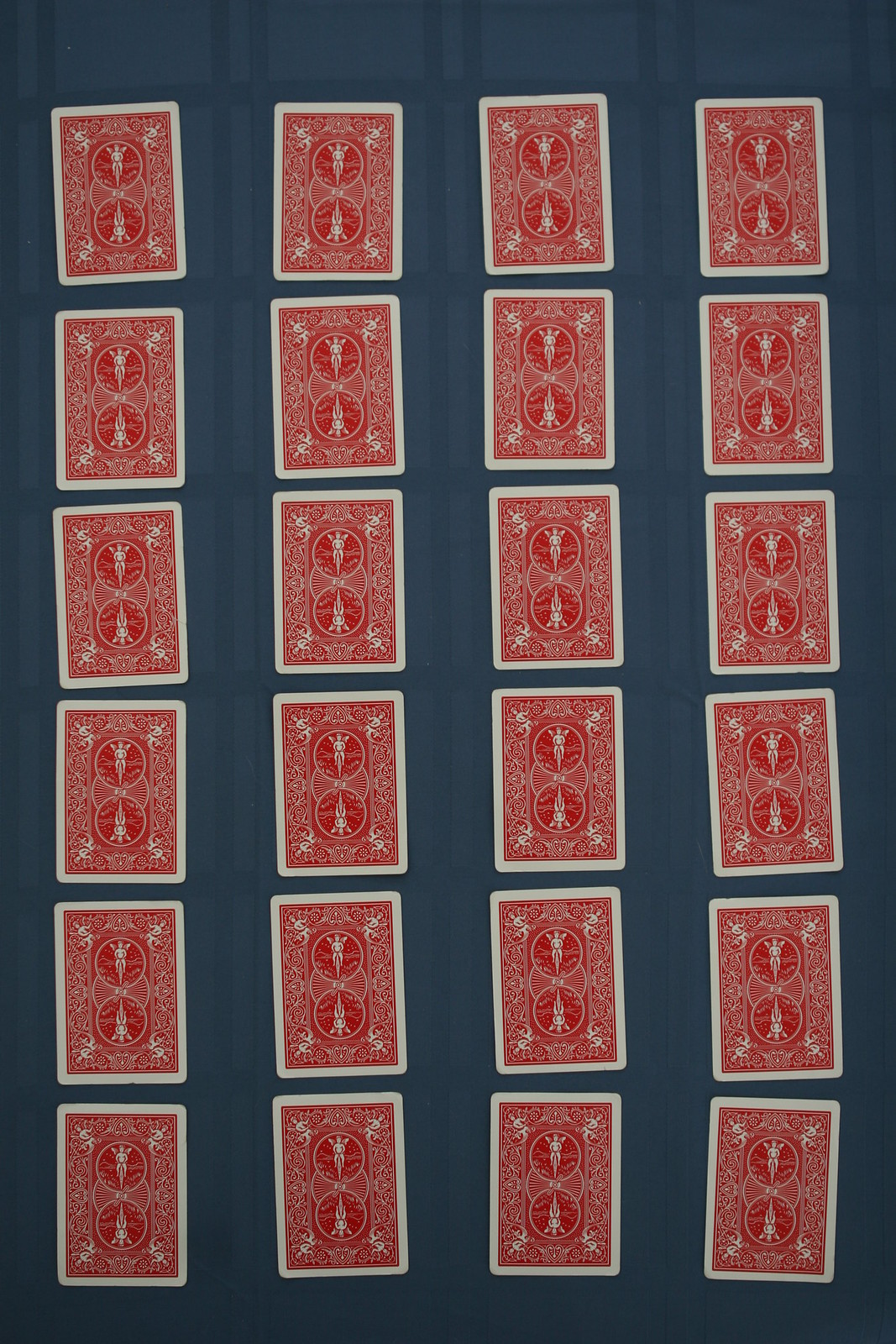The image features a background of blue tiles, which could be interpreted as a table, floor, cloth, or wall due to the ambiguous context. Laid out on this surface are 24 playing cards arranged in a grid of 6 rows by 4 columns. Each card is shown with its back facing up, displaying the iconic red and white design from the Bicycle Deck brand. The design on the back of each card depicts an angel riding a vintage bicycle, accompanied by merpeople in each corner. This design is mirrored, allowing it to be identically viewed regardless of the card's orientation. All the cards appear to be in pristine condition, suggesting they are either new or well-maintained. Although arranged in a grid, the cards are slightly misaligned, preventing perfect horizontal or vertical straight lines.